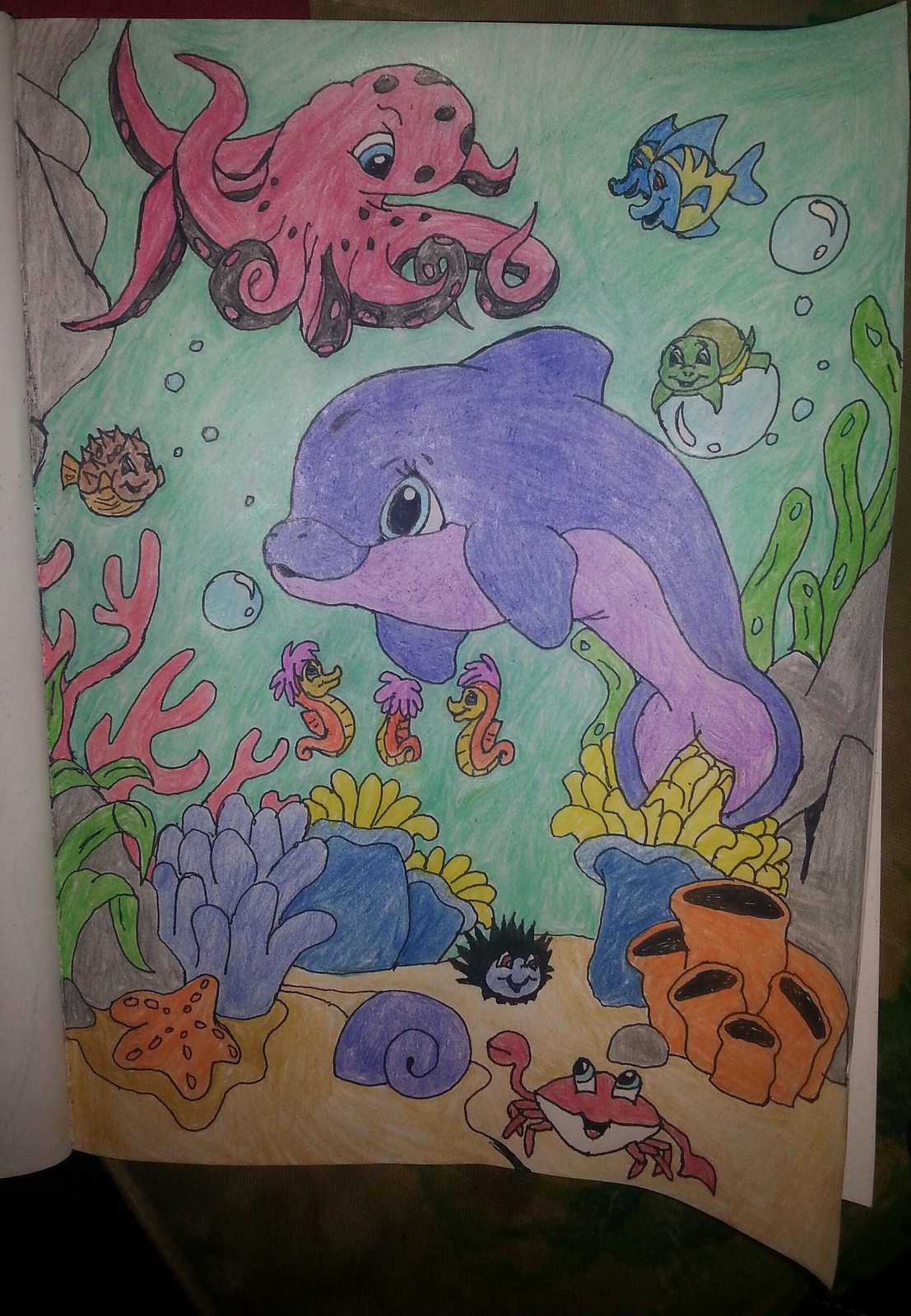This vibrant, hand-drawn underwater scene is teeming with life and detail, showcasing the whimsical creativity of a young artist. The picture features an array of marine creatures, including a playful dolphin, a curious octopus, a crab, various fish, seahorses, and a tiny turtle. The seafloor is dotted with colorful coral, starfish, and rocky formations, while the background is painted in a teal hue to represent the water. Bubbles are scattered throughout the scene, adding to the lively underwater ambiance. Despite the somewhat rough and swiftly executed coloring, the artwork captures the enchanting diversity of ocean life, making it a captivating piece full of movement and color.